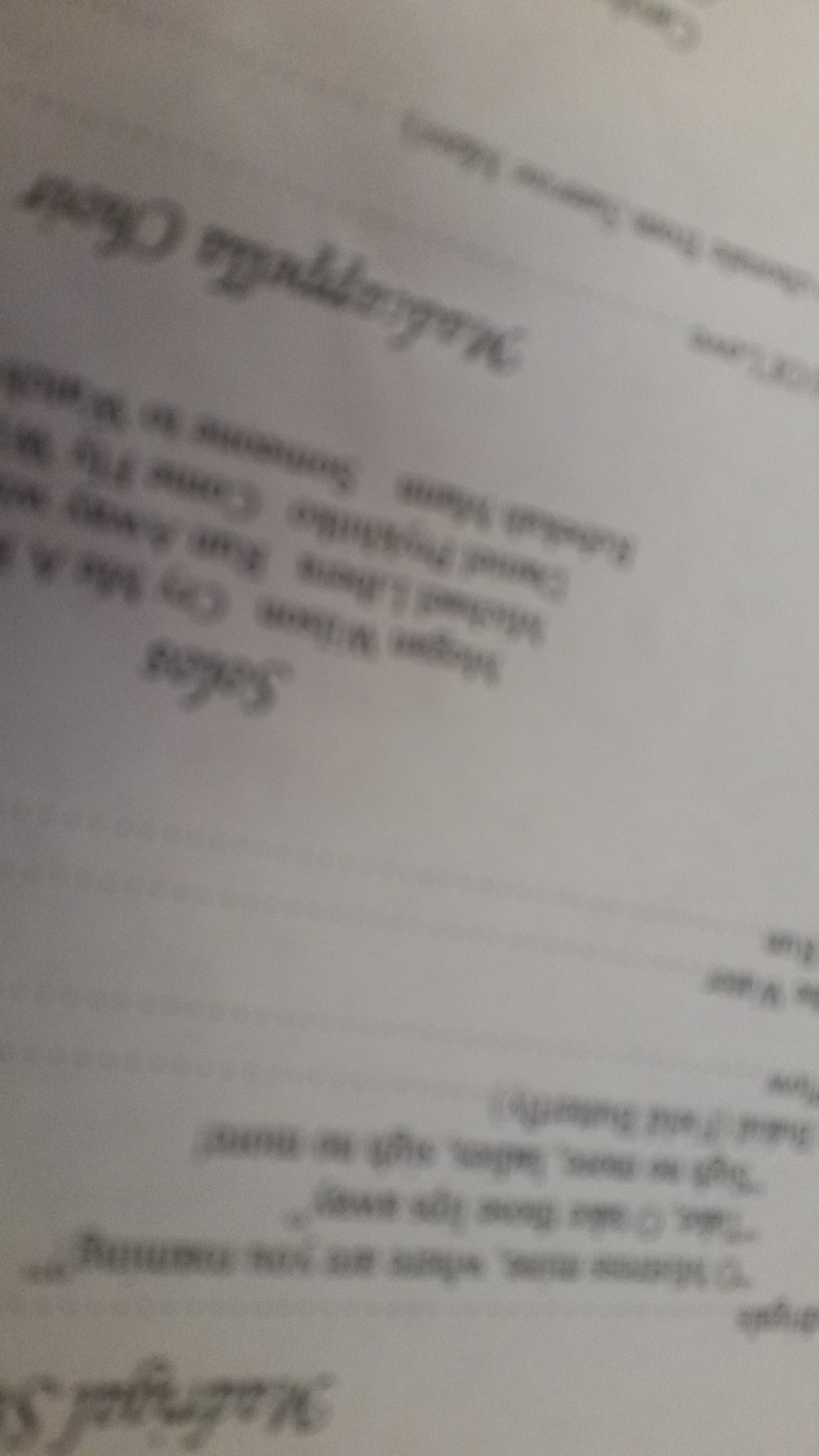In this image, there is an upside-down and blurry menu, making it difficult to discern the details. The menu is organized into three distinct sections. The middle section partially shows the word "Salads," and lists four different options underneath it. The top section appears to contain eight menu items, though the specifics are unclear due to the image quality and orientation.